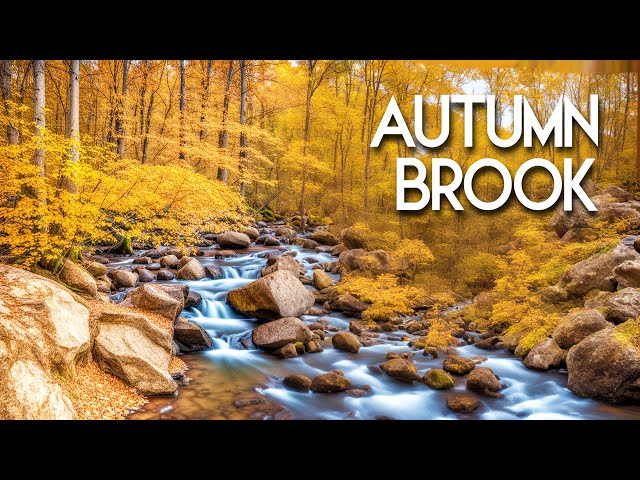The image is a detailed digital illustration, possibly AI-generated, depicting a serene outdoor scene in a dense forest. A light blue stream with a whitish glow follows a winding path towards the center of the image. The stream is flanked by numerous rocks of varying sizes, some of which are moss-covered. The foliage on the trees is yellow, evoking the colors of autumn. The dense woods create a rich, immersive setting. At the top right corner, white block text reads "Autumn Brook." The image features black letterboxing at the top and bottom, suggesting a weather and landscape-themed style, potentially used for a poster or promotional brochure.